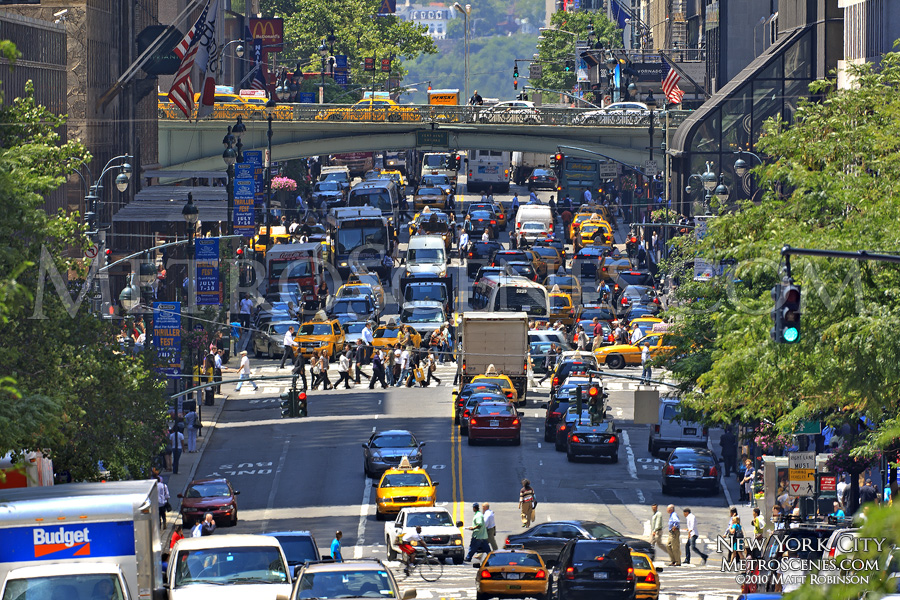This vibrant daytime photograph captures a bustling street in New York City, characterized by six lanes of traffic — three lanes going in each direction, separated by a yellow double line. The road descends a gentle hill, flanked by trees and partial views of buildings adorned with American flags. Amidst the heavy traffic, yellow taxi cabs and buses are prominent, along with a Budget truck visible in the lower left corner. Pedestrians traverse the street at various points, and cyclists weave through the crowd. A green traffic light on the right-hand side of the image signals the flow of vehicles. Street lamps dot the scene but remain unlit due to the daylight. In the background, a bridge filled with vehicles spans the width of the street. Detailed information in the lower right-hand corner of the image states, "New York City MetroScenes.com, copyright 2010, Matt Robinson." Far in the distance, trees and houses can be seen.